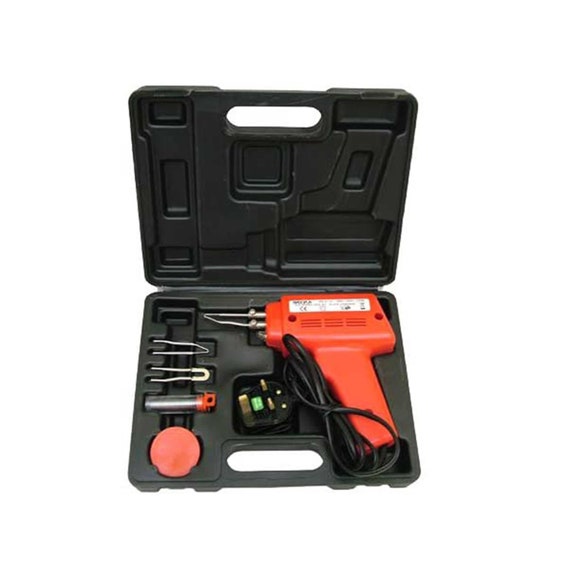The image depicts a neatly organized black hard-covered case open to reveal a red corded tool, which appears to be some sort of power tool. The case is designed with specific compartments to securely hold the tool and its accessories. The main compartment houses the red tool with a black cord, positioned on the right side. There are multiple silver-colored implements to the left, including several tweezer-like tools at the top and a straight silver rod below them. Additionally, there's a red circular attachment, possibly a buffer, located at the bottom of the case. The case also features a handle for easy carrying and the background of the image is a clean, well-lit white surface. The overall photograph is bright and clear, emphasizing the details of the tools and the case.